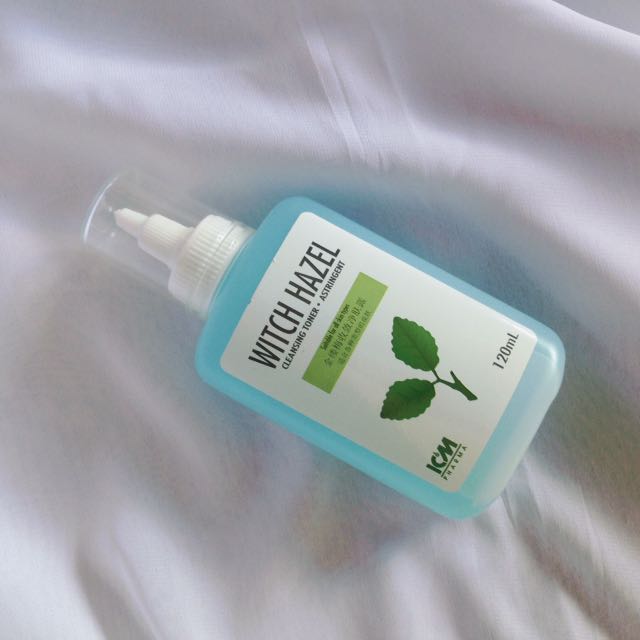This image features a close-up of a bottle of witch hazel resting at an angle on a piece of folded white fabric. The bottle is clear with a light blue or turquoise liquid inside, giving it a bluish-green appearance. It features a clear cap and a white nozzle top, designed for squeezing rather than spraying.

The bottle's white rectangular label prominently displays "Witch Hazel" in black font at the top. Below, "Cleansing Toner" and "Astringent" are printed, separated by a dot. A green box on the label, likely reading "suitable for all skin types," and a graphic of two rich green leaves add color and detail. The bottom left of the label features "ICM Pharma" (the brand name) or simply "ICM," while the bottom right indicates the bottle's volume as 120 milliliters. 

The background showcases a piece of white fabric, possibly a tablecloth, enhancing the clean and simple aesthetic of the image.